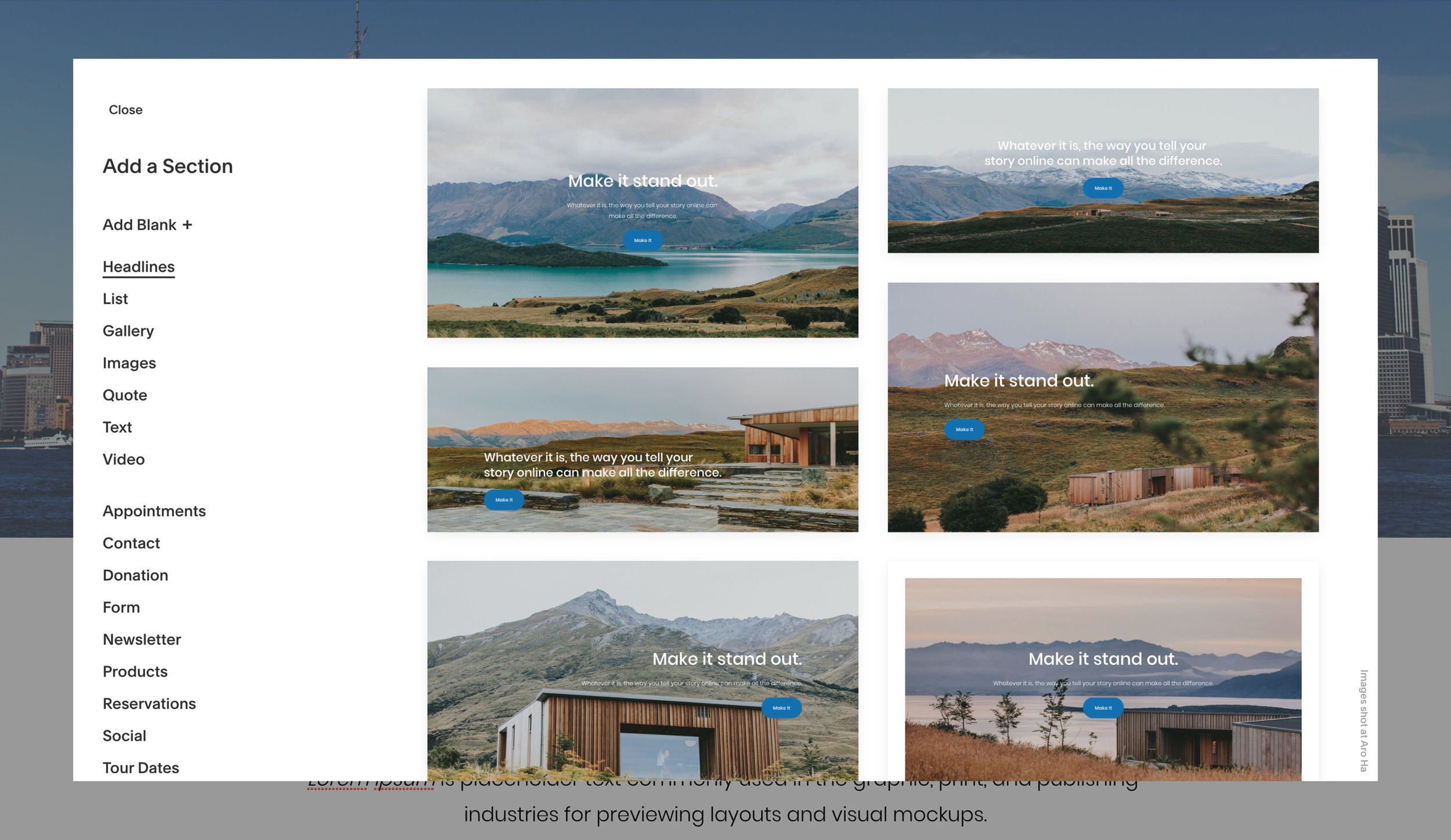This webpage features a gallery of six images, prominently displaying wooden structures that could be tiny houses, barns, or other buildings. The scenes are nestled within picturesque landscapes, often with mountains or lakes in the background. In the foreground, an overlay menu covers part of an image depicting a city. This menu is a large rectangle with a slightly larger rectangle behind it. In the left corner of the overlay, there is a "Close" button. Below it, in a larger font, is the text "Add a Section". Further down, in smaller font, it reads "Add Blank" accompanied by a plus sign. Following this is a list of options, each underlined by a black line: "Headlines," "List," "Gallery," "Images," "Quote," "Text," and "Video." Another space separates this section from additional options: "Appointments," "Contact," "Donation," "Form," "Newsletter," "Products," "Reservations," "Social," and "Tour Dates." The images in the gallery typically feature serene outdoor settings, some showcasing bodies of water, others highlighting rustic structures against the backdrop of nature.